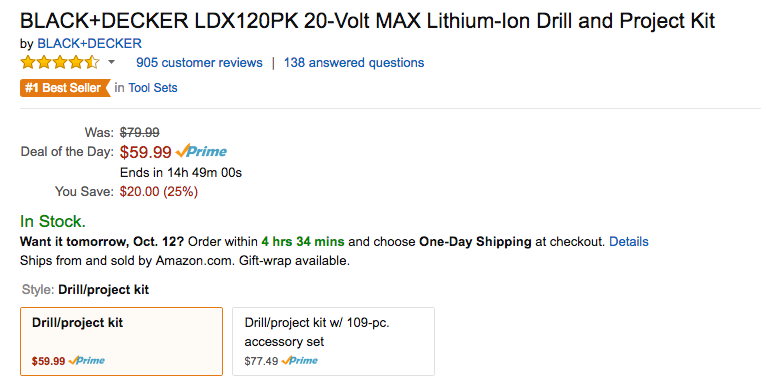This image displays a product listing page on Amazon for the Black and Decker LDX12PAC 20-Volt Max Lithium-Ion Drill and Project Kit. The product name, "Black and Decker," is highlighted in blue, indicating it is clickable for more information. The listing boasts a high customer rating of 4.5 stars based on 905 reviews and has 138 answered questions, reflecting its popularity and customer engagement.

Prominently featured is the label "Number 1 Best Seller in Tool Sets," highlighting the product's leading position in its category. Originally priced at $79.99, the item is available as the "Deal of the Day" for $59.99, offering a 25% discount equating to a $20 saving. The "Prime" badge next to the discounted price suggests expedited shipping for Prime members, with the promotion ending in 14 hours, 49 minutes, and 0 seconds from the time displayed.

The item is in stock, as indicated by the green "In Stock" status. For expedited delivery, customers are urged to order within 4 hours and 34 minutes to receive it by tomorrow, October 12th, via one-day shipping, with an option to click on "Details" for more information.

At the bottom of the page, there are options for different kit configurations, including a drill project kit and a gel project kit, each comprising 109 pieces.